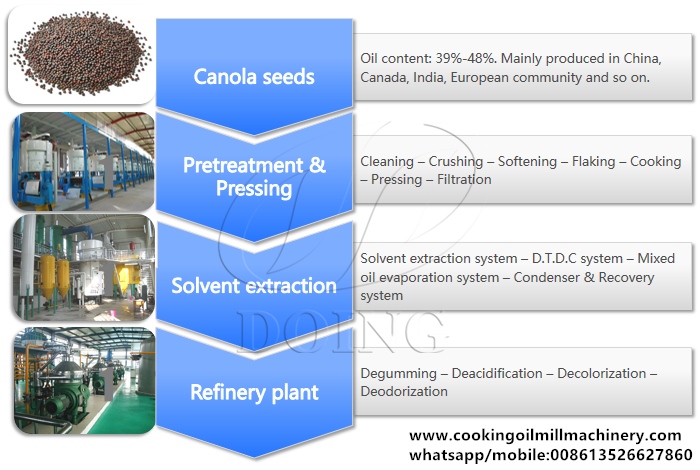This diagram presents a detailed overview of the canola oil production process across four sections. 

- At the top left, there is an image of a pile of canola seeds. Adjacent to this, “Canola Seeds” is prominently displayed in white text on a blue background. To the right, additional information is provided: oil content ranges between 39% to 48%, and it's primarily produced in China, Canada, India, and the European Community, among other regions.

- Below, the second image features a blue and gray processing machine or factory. Next to this, the label "Pretreatment and Pressing" appears on a blue background. Further right, additional details on this process are set against a gray background.

- The third section shows another machinery setup, characterized by yellow and gray colors. Beside this image, the term "Solvent Extraction" is highlighted. Additional relevant information follows to the right.

- At the bottom, the final image depicts a refinery plant, illustrated in greens and grays. The label to the right reads "Refinery Plant," followed by four words that start with the letter 'D,' all placed within a rectangular gray background. 

- A website link is positioned at the bottom of the diagram in black text. 

This comprehensive layout encapsulates the steps and key data points within the canola oil production process.